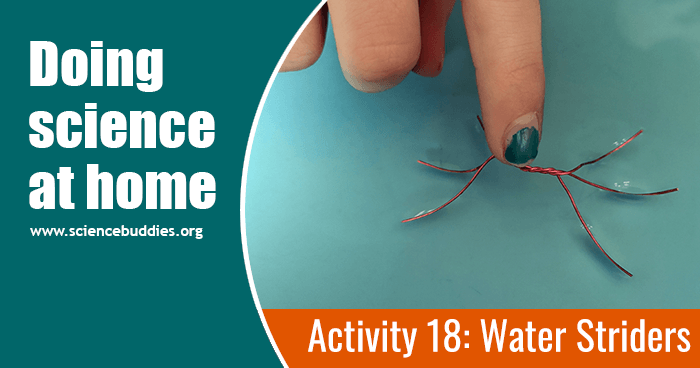The image features a green background that transitions from darker on the left to lighter on the right. On the left side, a teal section spans about a third of the image's width. This section is outlined on the right by a convex curve and contains bold, thick white text that reads "Doing Science at Home" in a mix of capitalized and lowercase letters. Beneath this, smaller white text displays the URL "www.sciencebuddies.org."

On the right side of the image, a close-up photo shows a partially visible hand with chipped teal fingernail polish pressing down on three intertwined copper wires. The wires appear to float on water, creating a distinctive surface tension effect observable in the water's bow around the intersections of the wires. An orange bar at the bottom of the image contains white text reading "Activity 18: Water Striders."